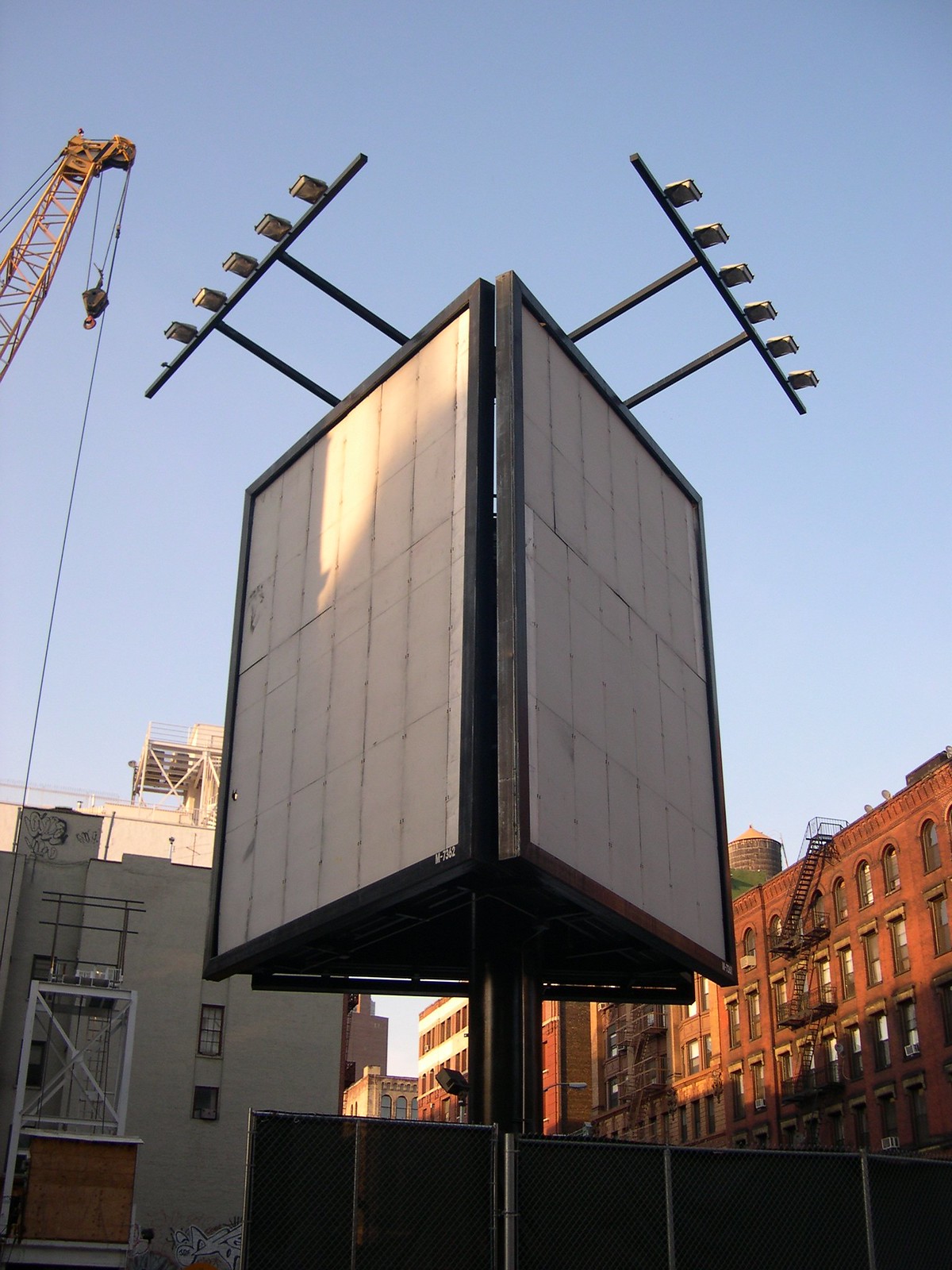This image captures a bustling downtown scene under a clear, sunlit sky. Central to the composition is a large, triangular billboard structure, completely devoid of any advertisements, revealing blank white surfaces on all visible panels. The billboard is equipped with numerous lights positioned on poles above it, presumably to illuminate it at night. Surrounding the billboard are several prominent buildings, notable among them a towering red brick structure on the right, adorned with rows of windows and fire escape ladders. A water tower perches on one of the rooftops, adding to the urban atmosphere. To the left, a tall white building with additional ladders or metal structures is visible. The upper left corner of the image features a yellow crane, its pulleys and chains slightly extending into the frame. The entire billboard is encased in a metal fence at its base, marking the boundary of this prominent cityscape element.